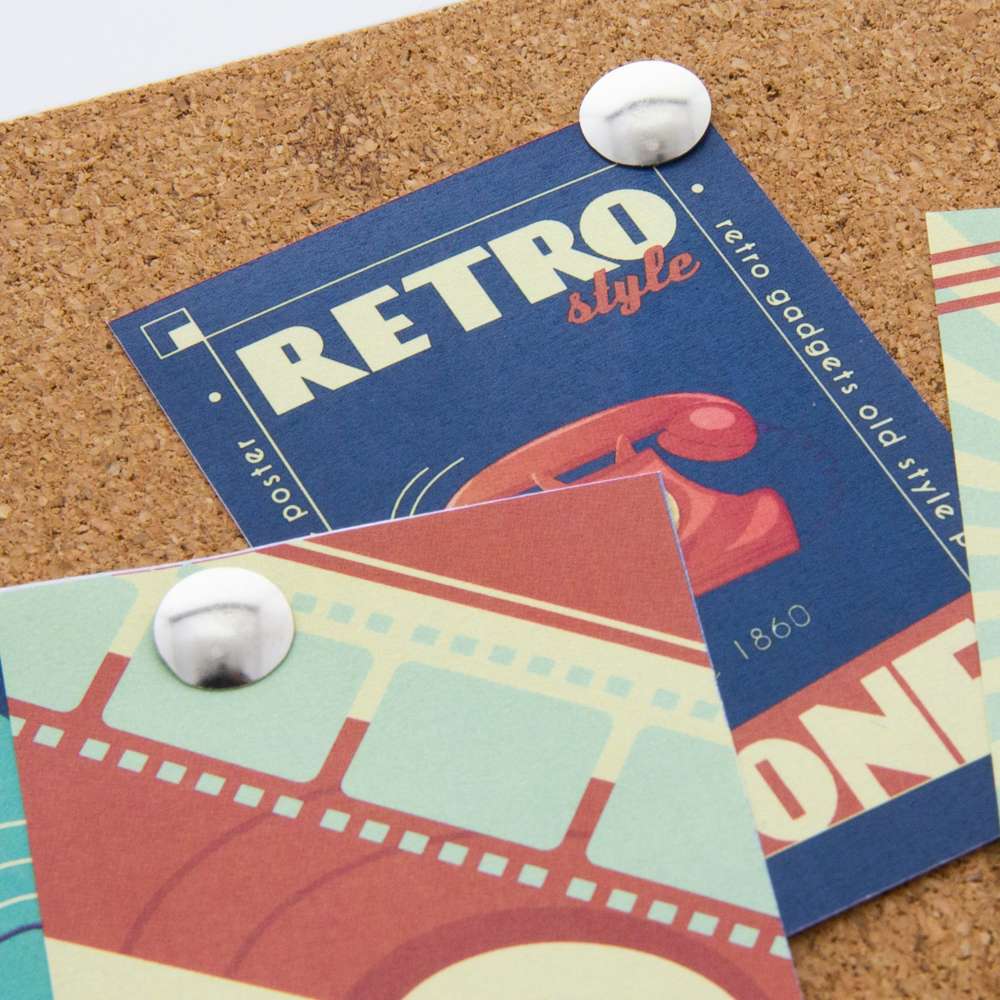The image depicts a brown, cork-textured surface adorned with multiple items pinned using silver push pins. Centered in the image is a blue book cover titled "Retro Style" in white text, featuring an old-fashioned red telephone prominently displayed, with the year 1860 written below it. Overlapping this central book cover on the bottom left is a postcard with a greenish-blue and red design, reminiscent of old camera films with small square holes. To the right of the "Retro Style" book cover, another card or poster is partially visible, adding to the nostalgic theme suggested by the arrangement. The detailed composition of books and postcards pinned to the corkboard captures a vintage aesthetic unified by the recurring use of retro imagery and colors.